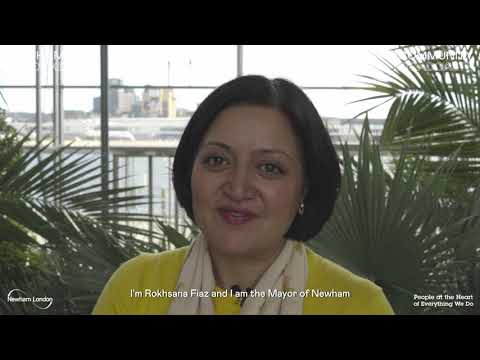A light-complected woman with short black hair is pictured wearing red lipstick and a yellow shirt, accessorized with a light cream-colored scarf. She is speaking into a microphone labeled "R-o-k-h-a H-s-a-n-s F-l-a-z" and identifies herself as the mayor of Nottingham. The photograph, which has poor resolution, shows a scene behind her where you can see plants and palm trees outside a window. There is text in the right corner that reads "Principal *something* of everything we do." On the left side, it vaguely states "Nottingham, London." The image features black strips at the top and bottom, making the photograph appear smaller within the space. In the background, beyond the greenery, you can see what seems to be water and a distant cityscape with a few high-rises and an indiscernible white object.